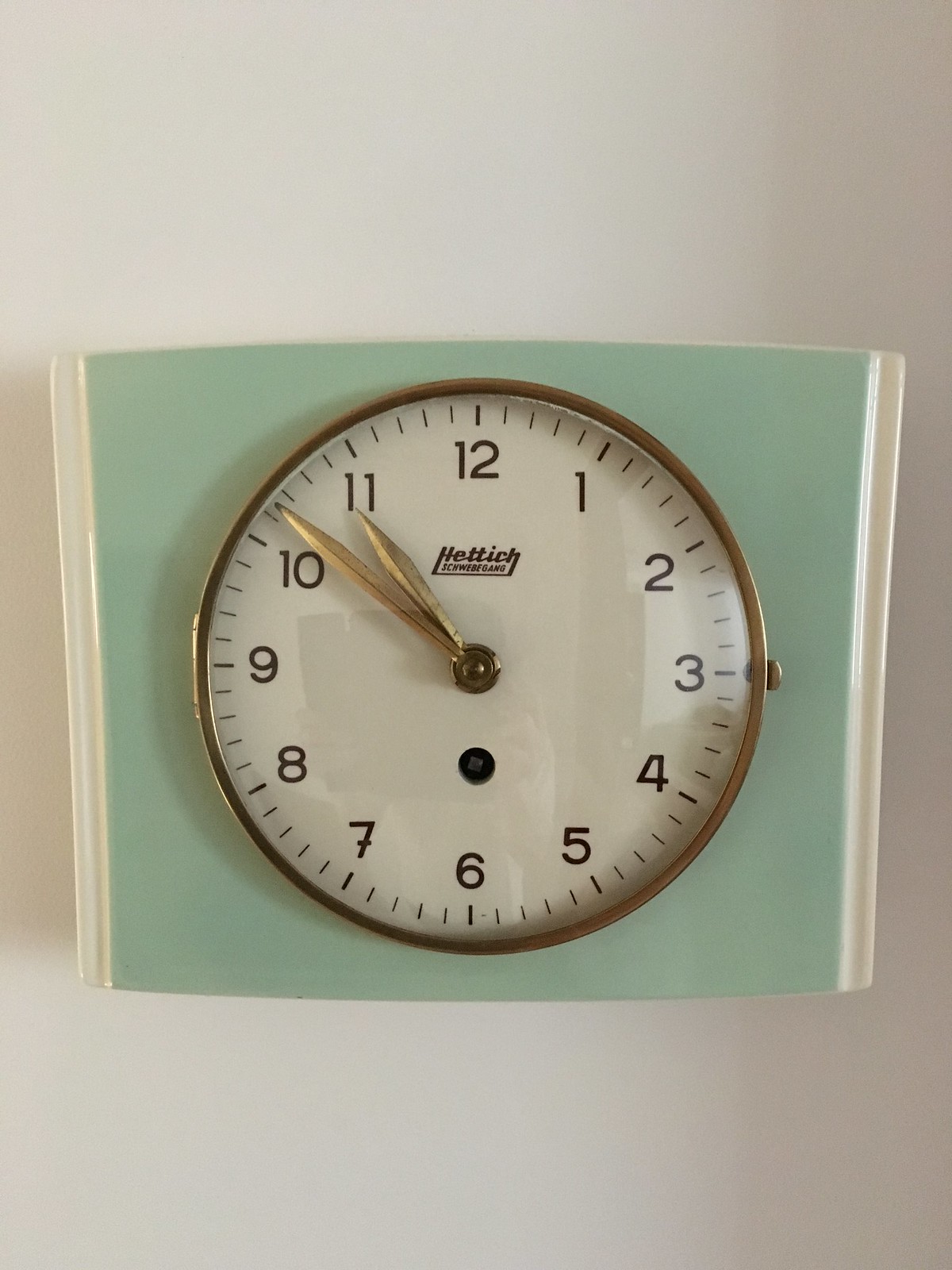Caption: 

A close-up of a round analog clock mounted on a plain white wall. The clock features brass hands pointing to approximately 10:52. The face of the clock is minimalist, with no additional graphics, and the numbers one through twelve are spelled out clearly. The clock's surrounding frame is light green and is accented by two white borders, adding a subtle touch of color to the otherwise stark setting.